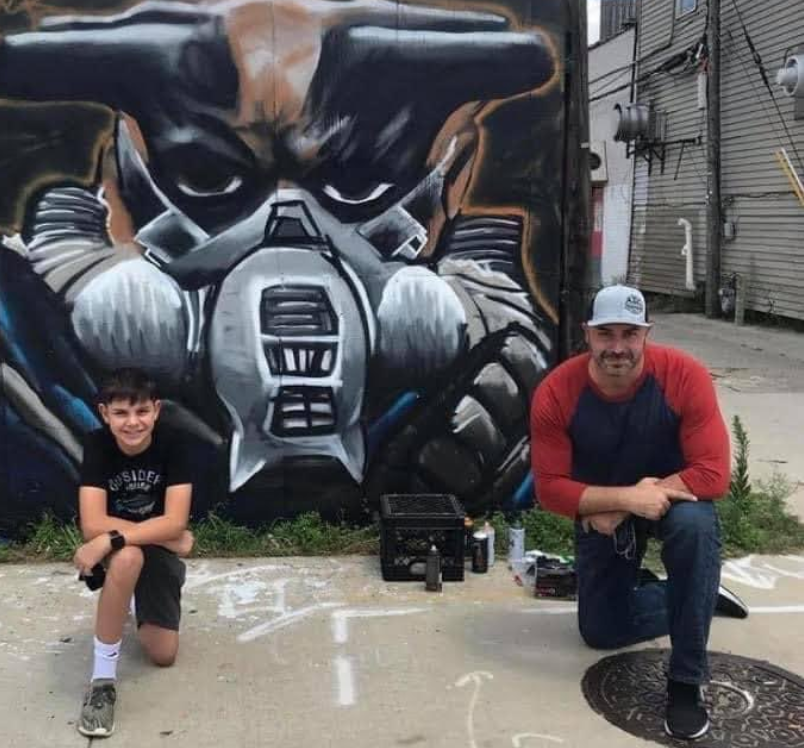The image captures what appears to be a father and son, kneeling on a pavement in front of a graffitied wall they seem to have worked on together. The boy, approximately 12-14 years old, is positioned on the left with his left knee on the ground and his right knee up, arms crossed over his upright knee. He is dressed in a black shirt, black shorts, white high top socks, and gray sneakers. About three or four feet to his right, the man, presumably his father, mirrors the boy's pose but with opposite legs positioned similarly. He wears a gray baseball cap, a red and blue long-sleeve Henley top, blue jeans, and black sneakers. Both have similar darker-than-white skin tones, suggesting a familial relation. Behind them, a vibrant graffiti mural featuring what appears to be a masked bulldog or possibly a dog driving a motorcycle adorns the wall, indicating their artistic handiwork. On the ground near the wall, a black milk crate and several spray paint cans lie, reinforcing the idea that they have recently completed the artwork.